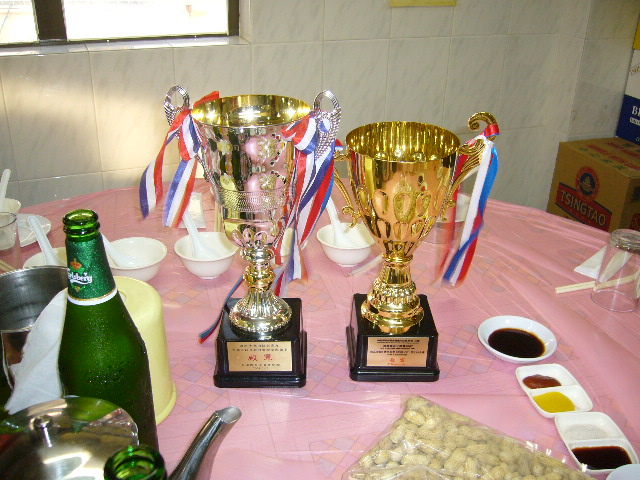Displayed on a round table draped with a pink, semi-transparent tablecloth, this image features two elegant trophies as its focal point. The larger trophy on the left is a silverish gold goblet, while the slightly smaller one on the right is fully gold. Both trophies are adorned with red, white, and blue ribbons hanging from their curved handles. They sit on a black wooden stand, centered on the table. Flanking the trophies are several white bowls and dishes, some containing different colored sauces, and others resembling ice cream or soup bowls with large spoons beside them. To the left of the trophies rests a green bottle, possibly liquor or beer, identifiable by its green label. Additionally, a silver tea kettle can be seen in the lower-left corner. In the foreground, a plastic bag filled with dry roasted peanuts is visible, along with an upside-down glass. The background features a marble wall and a window in the upper left corner, along with a Tsingtao-branded brown box on the right. The combination of decorative and functional items creates a rich, varied scene, blending celebratory and culinary elements.